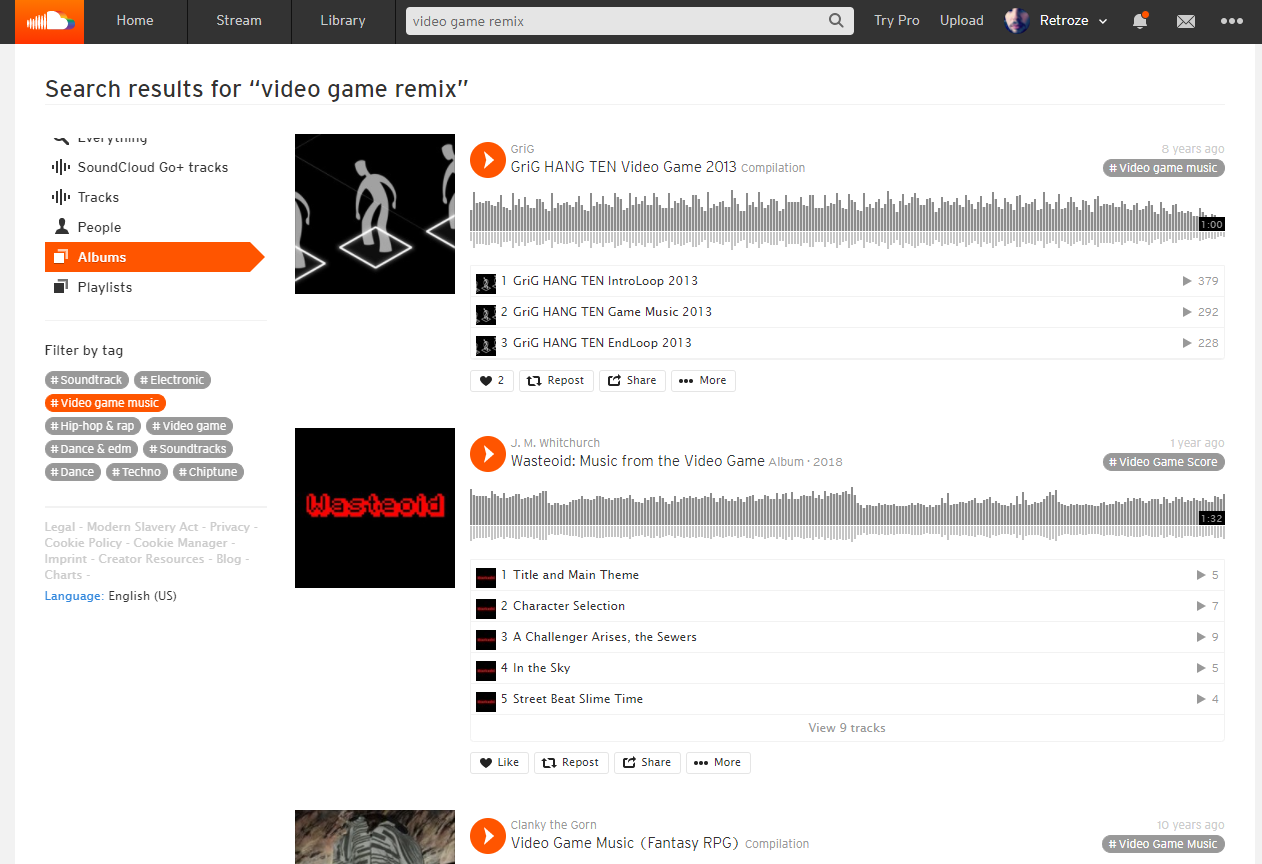A screen capture displays the search results for "video game remix" on the SoundCloud website. The image features small thumbnail images of album covers related to video game remixes. The primary navigation bar at the top includes the SoundCloud logo, along with options such as Home, Stream, Library, Search Bar, Try Pro, Upload, and Reference. The background shows a design of clouds, reinforcing the platform's branding. From this search, users can choose any of the displayed albums to listen to. However, to access all features, one might need to explore SoundCloud Go, the platform's premium service.